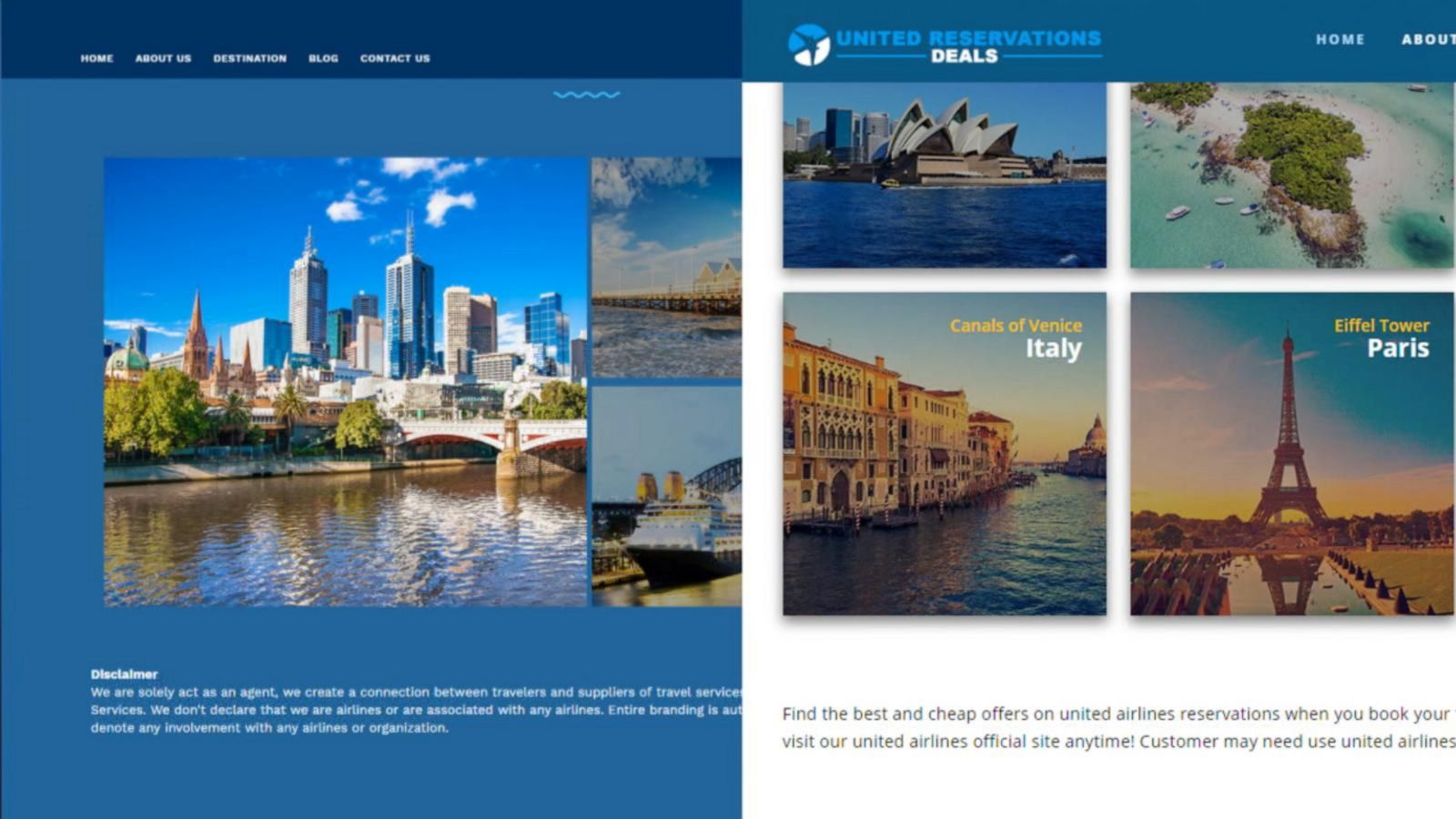The image comprises two screenshots from a website dedicated to United Reservations Deals. 

The right-hand screenshot prominently features the United Reservations Deals logo situated in the top-left corner within a blue box. Adjacent to the logo, the navigation bar includes options for "Home" and "About," although subsequent sections are not visible. The main content advertises various travel destinations. At the center, there is a picture of the Sydney Opera House. To its right, there’s an image of a tropical island. Below these, a photograph of the canals of Venice, Italy is displayed on the left, and to the right, an image of the Eiffel Tower with overlay text that reads "Eiffel Tower" in yellow and "Paris" in white. The background of the website is primarily white, and a promotional text at the bottom reads: "Find the best and cheap offers on United Airlines reservations when you book your visit our United Airlines official site anytime. Customer may need to use United Airlines."

The left-hand screenshot shows a section of the same website with a navy blue top bar. The navigation options here include "Home," "About Us," "The Nation Blogger," and "Contact Us." Below this, there is an image of a cityscape viewed from across a river, suggesting a port city, though the view is partially obscured. The bottom section features a white disclaimer text on a blue background, stating: "Disclaimer, we are solely act as an agent. We create a connection between travelers and suppliers of travel services." The text continues but is cut off, mentioning that the site does not claim to be affiliated with any airlines and clarifies its role as a travel agent. The remaining message is truncated but implies a further disassociation with any specific airline or organization.

Together, these screenshots provide an overview of the United Reservations Deals website, highlighting its promotional travel content and disclaimers regarding its role as an intermediary in travel services.